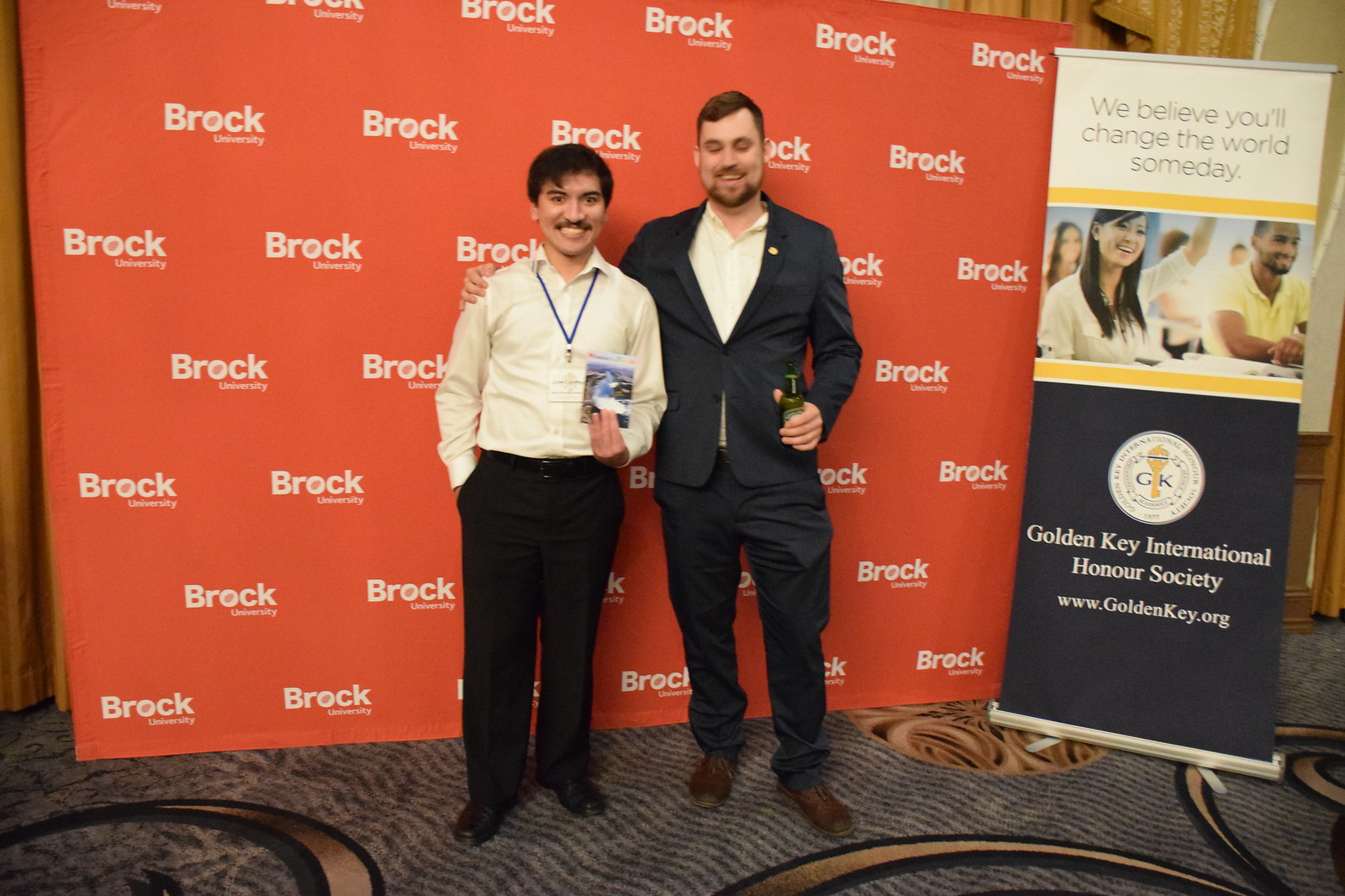In this photograph, two men are standing on a carpeted platform against an orange backdrop adorned with the Brock University logo pattern. To the right of the men, there is a sign for the Golden Key International Honor Society, bearing the slogan, "We believe you'll change the world someday." Both men appear to be affiliated with this honor society.

The man on the left has medium-length black hair, a black mustache, and is smiling broadly. He is wearing slacks and a white button-down shirt, with a lanyard around his neck. He holds up a small postcard or pass.

The man on the right, who is taller, has brown hair and a light beard. He is dressed in a blue suit without a tie and brown shoes, holding a Heineken bottle. The setting hints at an indoor event or function hosted by Brock University in collaboration with the Golden Key International Honor Society.